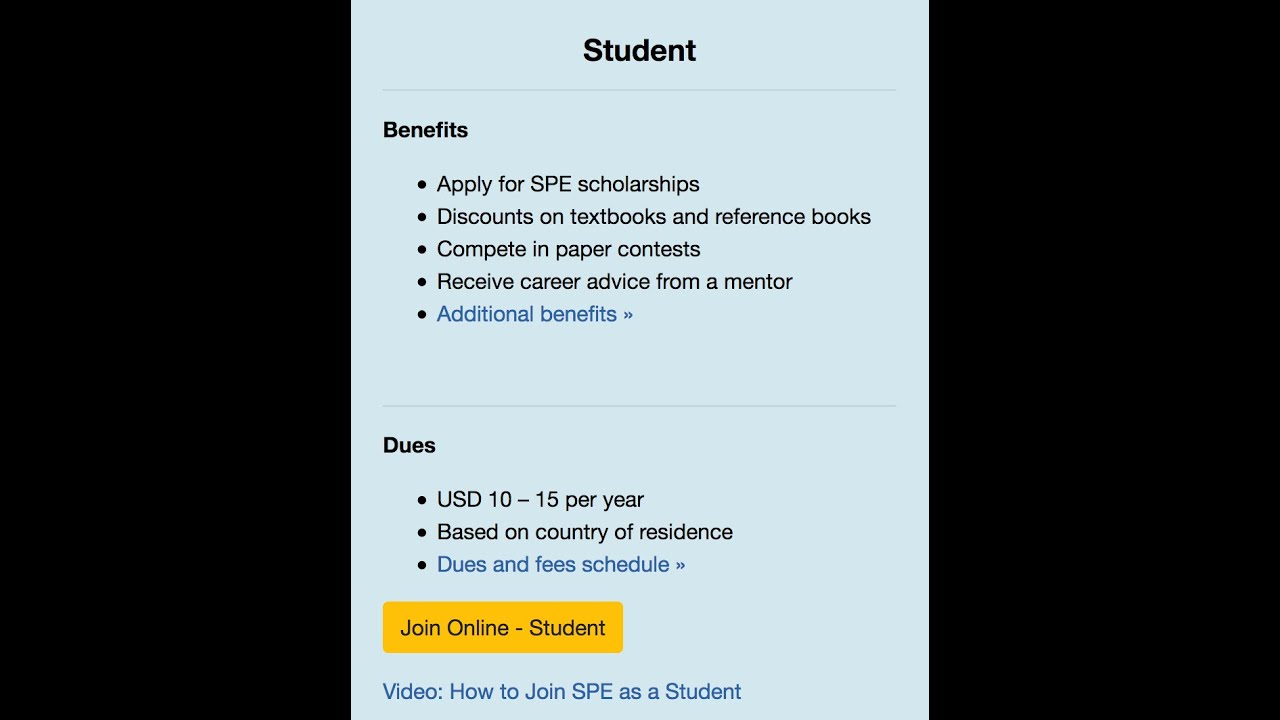The image features a predominantly black rectangle with a vertical blue stripe running down its center. On either side of the stripe, there are narrow black stripes accentuating the design. 

At the top of the blue stripe, the word "STUDENTS" is prominently displayed in large, bold print. Directly beneath this title, there's a faint line followed by the heading "Benefits." Under this heading, a list of bullet points outlines various advantages available to students:
1. Apply for SPE Scholarships
2. Discounts on textbooks and reference books
3. Compete in paper contests
4. Receive career advice from a mentor
5. Additional benefits (highlighted in a light blue font)

A horizontal line divides this section from the next, which is titled "Dues" in bold, dark font. Below, three bullet points provide further details:
1. USD 10-15 per year
2. Based on country of residence
3. Dues and fee schedule

Further down, there's a yellow button labeled "Online-Students," and at the very bottom of the image, there's an instructional prompt that reads "Video: How to join SPE as a student."